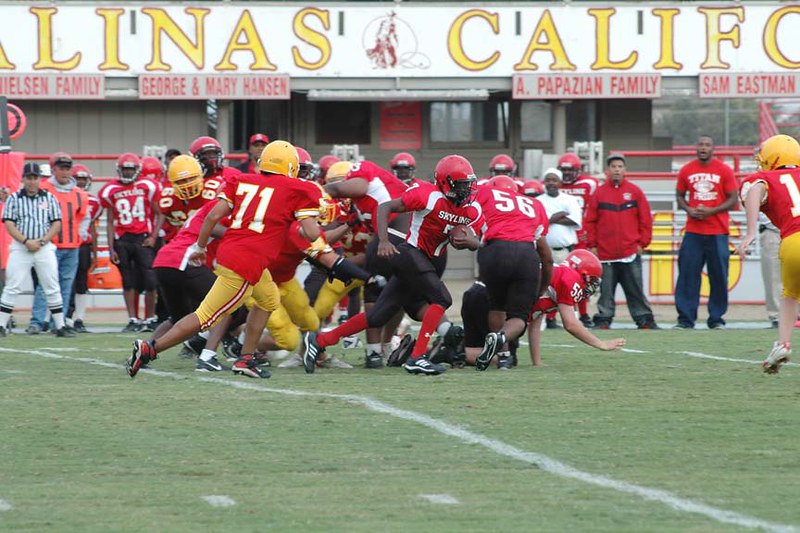This image depicts a bustling American football game on a vibrant green field marked with white lines. The players, clad in red jerseys, are divided into two teams: one team wears black pants and red helmets, while the other team sports gold pants and gold helmets. A dynamic huddle is unfolding amidst this clash, with some players seemingly tackled to the ground. In the background, a partially visible white banner with bold, yellow letters spells out "L-I-N-A-S" and "C-A-L-I-F-O," though the ends are cut off. Beneath the banner, a series of gray signs with red lettering are displayed, listing names: "Nelson family," "George and Mary Henson," "A. Papazian family," and "Sam Eastman." On the sidelines, a referee oversees the action, and a man in a red shirt emblazoned with "Titans" appears to be yelling, adding to the intensity of the scene.